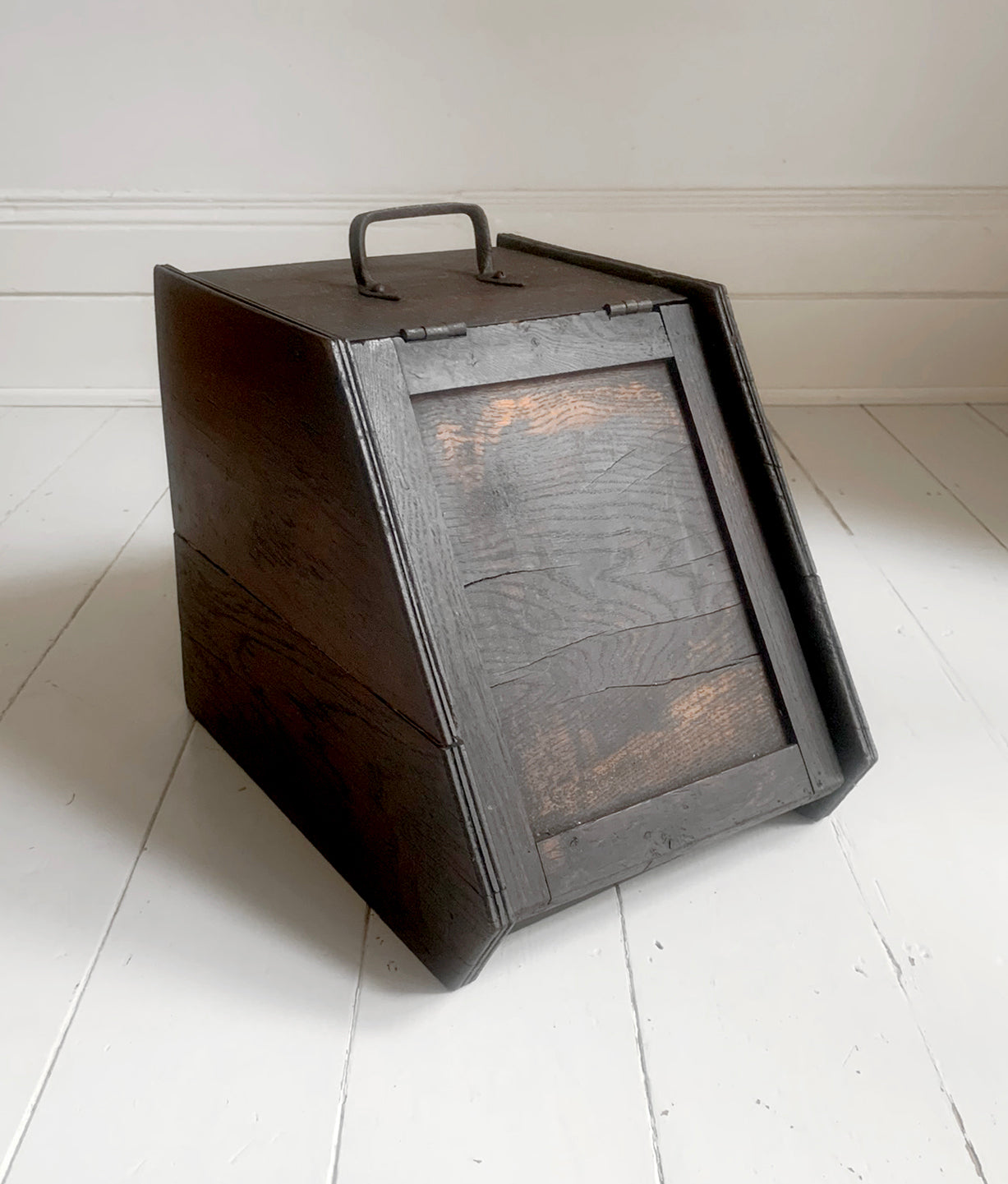In this photograph, a large antique wooden box is the focal point, set against a stark white wall and resting on a pink-painted wooden floor. The box is constructed from dark-stained mahogany wood, showcasing both lighter and darker areas that indicate age and wear. The front of the box features a hinged flap that lifts open, likely designed for storing bread, giving it the appearance of an old-fashioned bread box. The box’s unique structure is slanted, triangular at the front and square at the base, with the flap angled at about 45 degrees. A brown metal handle is mounted on the top, suggesting it can be carried to different locations. The box's weathered look is further evidenced by visible cracks and wear on the wood, reinforcing its vintage charm.